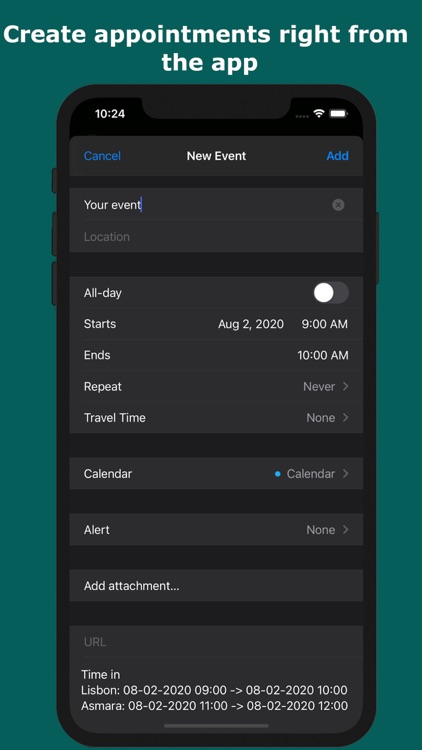This is a detailed graphic design illustration of an older model iPhone screen, showcasing various functional elements and interface components. 

The iPhone is depicted from the top view, making visible the volume buttons and silent switch on the left side, and the power button on the right. Notably, this model features a top-centered camera notch, rather than the isolated island design found in more recent versions. 

The primary background color of the interface is black. At the top-right corner of the screen, you can spot the Wi-Fi and battery status icons, while the top-left shows the time, 10:24, all rendered in white text.

The main content of the screen displays the "New Event" creation window from the Calendar app. In this window, the text "New Event" is centered in white. On either side of this header, there are interactable options in blue text: "Cancel" on the left and "Add" on the right. Directly below the header, a blue cursor indicates where event details can be typed, with a grayed-out "Location" field underneath.

Next is a section with several options: "All Day" with an adjacent toggle switch; "Starts," "Ends," "Repeat," and "Travel Time." 

Below this section, there is an expandable "Calendar" option, denoted by an arrow pointing to the right, indicating that users can select a specific calendar for the event. Further down, an "Alert" option set to "None," which is also interactable, allowing users to set reminders. 

Additionally, there is an "Add Attachment" option, followed by a text input field for adding a URL. Finally, at the bottom, there is a section labeled "Time In," which seems dedicated to automating or indicating the schedule for the event or activity.